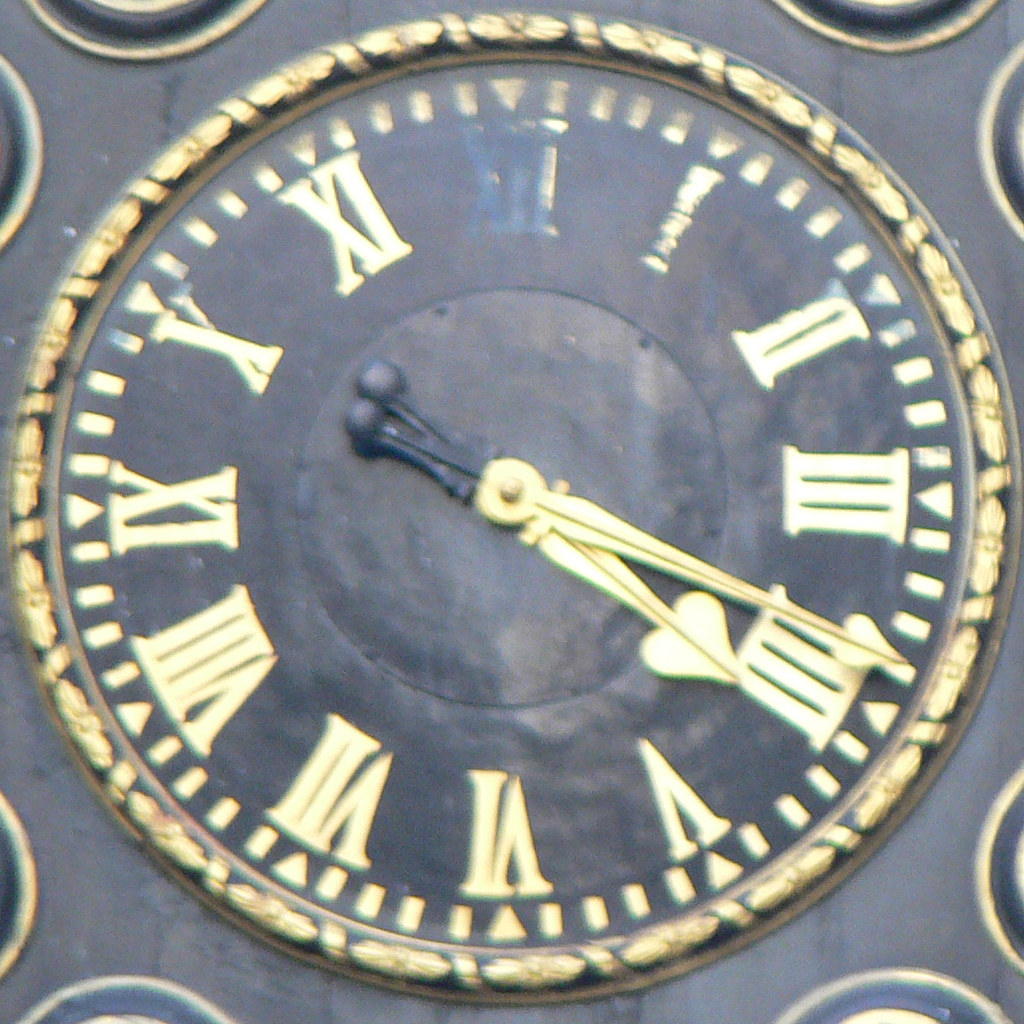This photograph captures a slightly blurry, close-up view of an analog clock face with a round, black face that appears slightly weathered and possibly metal. The clock is illuminated by natural sunlight, suggesting it is outdoors. It features gold Roman numerals, though the numeral for 12 is notably worn off, leaving just traces of gold. Surrounding the clock face is a gold border composed of elliptical symbols separated by vertical bars. The gold hour and minute hands are shaped like daggers with black handles and end in small sphere shapes, almost resembling hearts. The clock is displaying the time as fourteen minutes past four. Earnest about details, minute marks are also visible around the edge of the face.